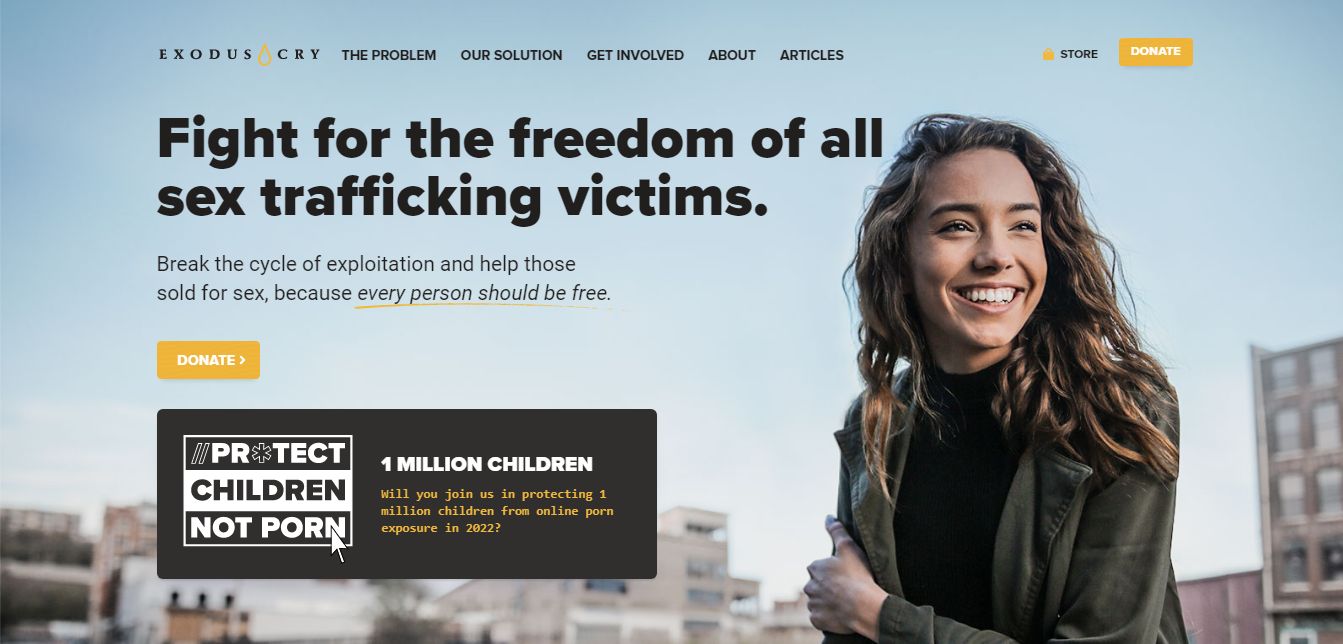This image showcases a webpage belonging to the charity organization Exodus Cry, dedicated to combating sex trafficking. The top-left corner prominently features the Exodus Cry logo, and the navigation menu includes options such as "The Problem," "Our Solution," "Get Involved," "About," and "Articles." Dominating the page is a powerful message in bold black text: "Fight for Freedom of All Sex Trafficking Victims. Break the cycle of exploitation and help those sold for sex because every person should be free." 

Beneath this call to action, a prominent orange "Donate" button invites visitors to contribute to the cause. Adjacent to it, a symbol with the phrase "Protect Children, Not Porn" urges visitors to join the effort in safeguarding one million children from online porn exposure in 2022.

In the top-right corner, icons for a store and another donation option provide additional ways to support the organization. The cursor on the page appears to be clicking on the "Protect Children, Not Porn" symbol.

The background of the webpage features a city skyline with a young Caucasian girl pictured from the waist up, smiling and gazing to the left. She wears a dark greenish jacket over a black shirt, has slightly longer than shoulder-length brown hair, tan skin, and noticeably white teeth, exuding a hopeful and positive demeanor.